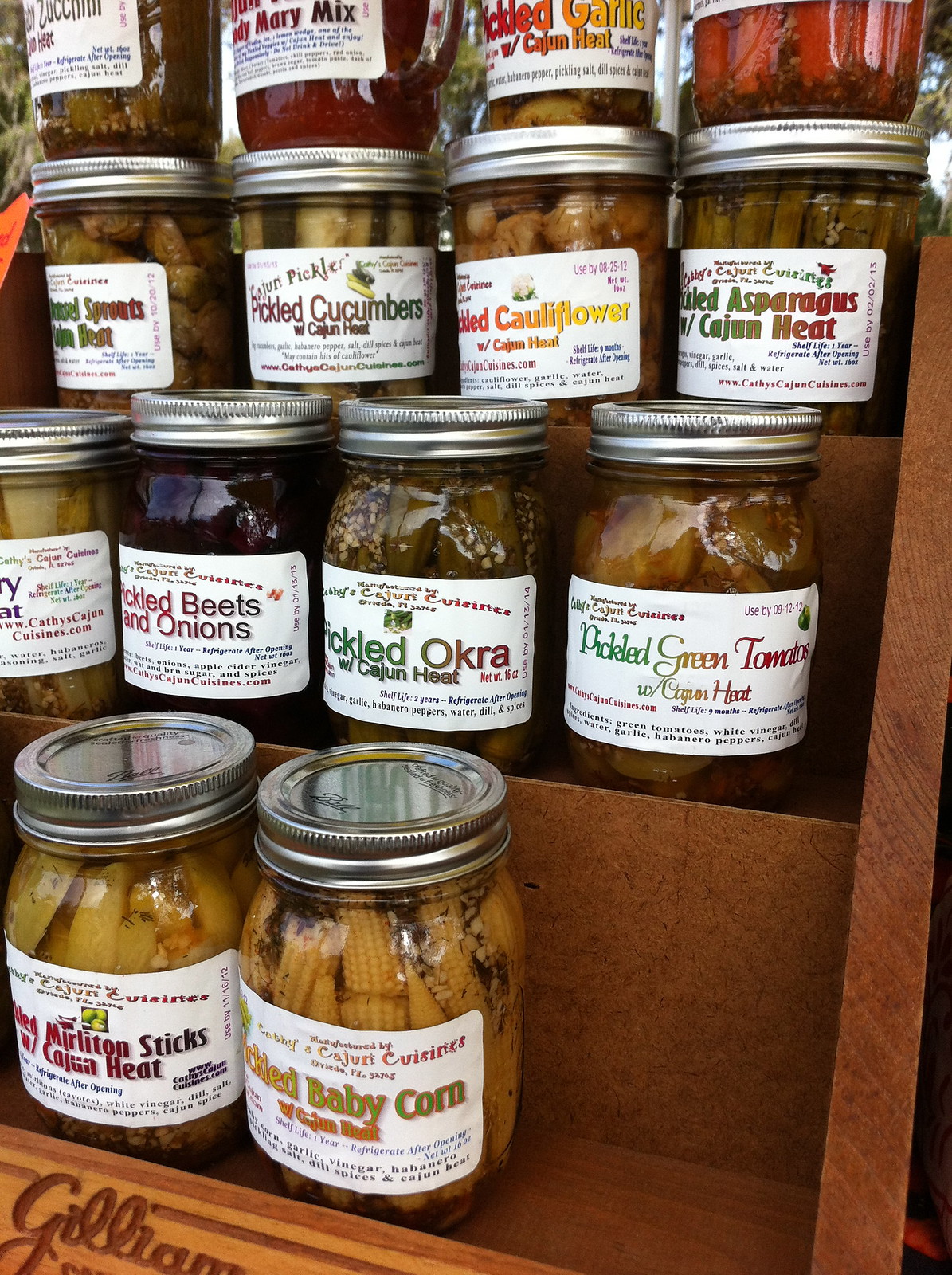This vertical rectangular image captures a display in a specialty or local grocery store, showcasing an assortment of canned vegetables on a rustic, brown wooden shelf. The display features approximately 14 jars, each with a silver twist cap, resembling typical pickle jars, likely around 16 ounces in size. The jars are meticulously organized in three rows, though the top row includes some jars stacked atop others. The white labels on the jars display a variety of colorful titles, revealing contents like baby corn, pickled green tomatoes, pickled okra, pickled beets with onions, asparagus with Cajun heat, pickled cauliflower, and pickled cucumbers with Cajun heat, among others. At the bottom of the display, the name "Gilliam" is carved into the wood, hinting at a small farm or local producer rather than a chain company. One noticeable detail is an empty space on the very bottom row, adding to the authenticity of the display.